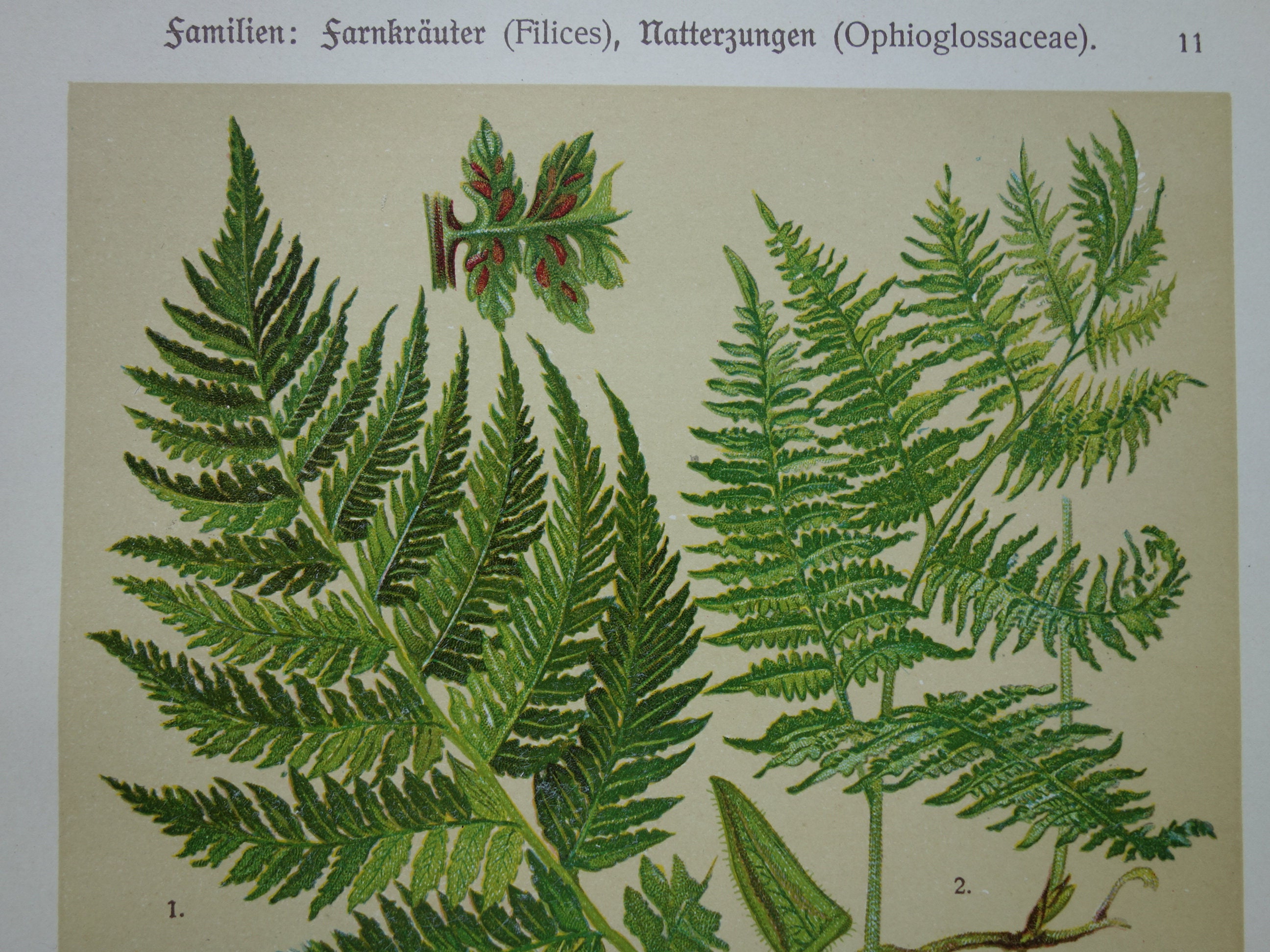The image depicts a green fern plant against a gray background, taken from what appears to be a botanical book or textbook. The title at the top is in a foreign language, reading "Familian Farnkrauter (Frlilcs Natterzungen, Ophioglossaceae)." The fern features a long stem with multiple narrow leaves, each culminating in a sharp and pointy tip. Some of the leaves exhibit a touch of brown, likely indicating seeds. The fern resembles common varieties, with some leaves displaying fancier curls along the edges, suggesting different species or varieties within the Ophioglossaceae family.